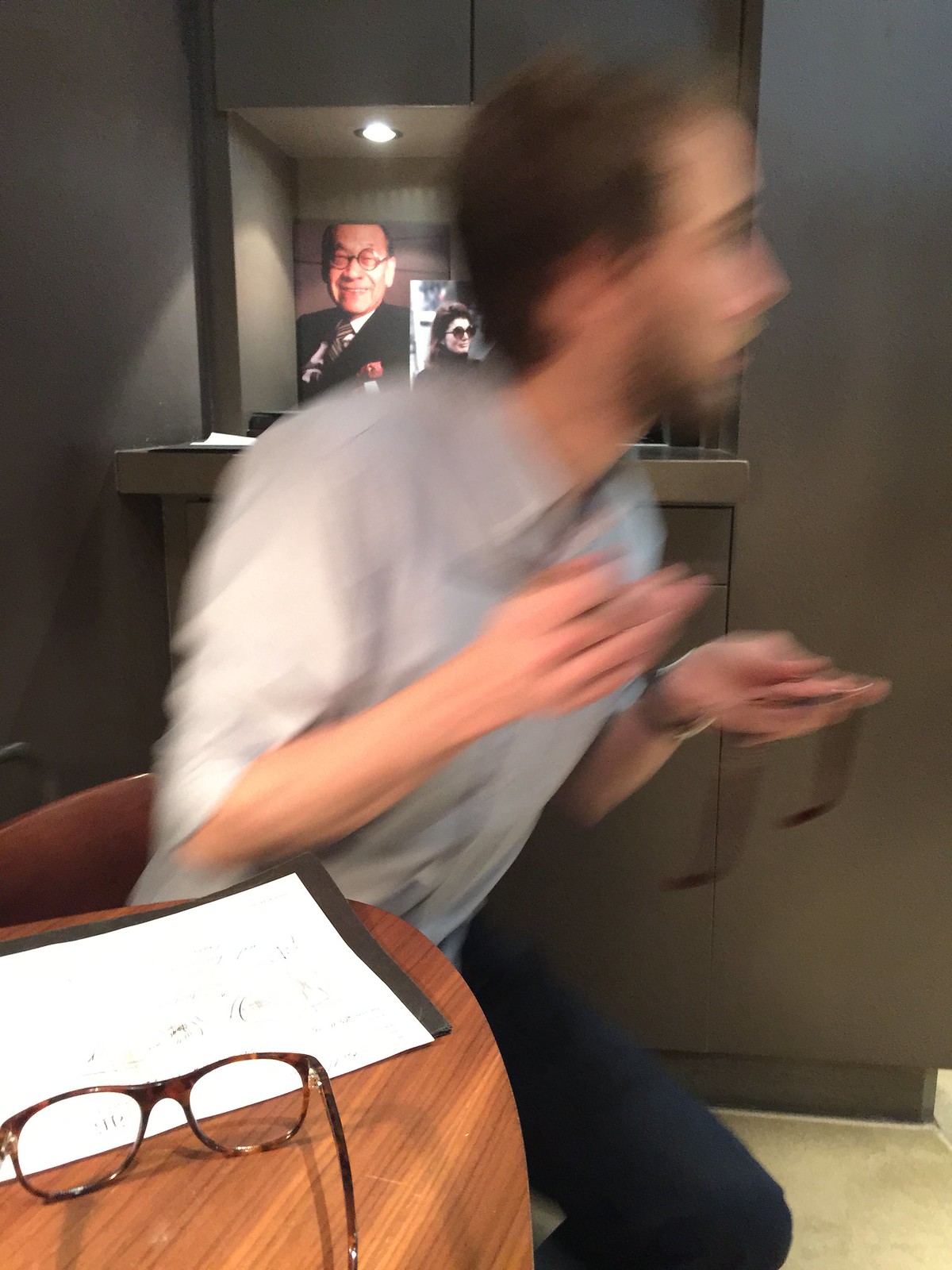In this motion-blurred image, a man in his mid-twenties appears to be rapidly standing up from a rounded, wooden table, his image filed with kinetic energy. He's wearing a brown (or possibly gray) short-sleeve shirt and blue jeans. The blur suggests vigorous movement, capturing him in an almost transitional state between sitting and standing. His torso is twisted towards his left, revealing his arm and the side of his face, both slightly obscured by the motion. His left hand seems to be holding a pair of glasses, resting on the table, next to a couple of pieces of paper - one white and one black, possibly with some writing on them. The table also hosts another set of reading glasses with their arms facing away. In the dark gray background, there are two photographs hanging on the wall: one of an older Asian man with round glasses and another of a woman in dark sunglasses. The floor beneath the scene is an industrial-looking Formica with a yellow tint.